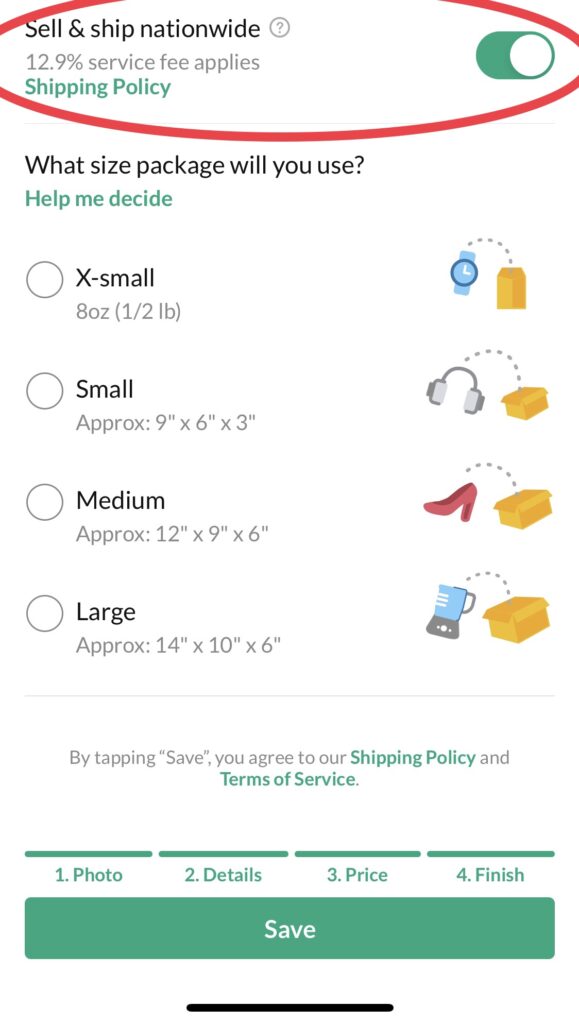### Detailed Caption:

The image depicts the checkout page of a shipping company's website, focused on order shipping details. At the top, a red circle highlights a notification that reads, "Sell and ship nationwide, 12.9% service fee applies." Adjacent to this notification is a green button labeled "Shipping Policy," which has been activated as indicated by the green slider bar on the right.

Below this section, the page displays text that says, "What size package will we use?" Next to it, in green text, there's a clickable link labeled "Help me decide." 

The interface offers four size options for packaging, each represented by a dot:
1. **Extra Small (8 ounces, or half a pound):** Illustrated with an image of a watch.
2. **Small (Approximately 9 x 6 x 3 inches):** Represented by a pair of headphones.
3. **Medium (Approximately 12 x 9 x 6 inches):** Depicted with a pair of shoes.
4. **Large (Approximately 14 x 10 x 6 inches):** Shown with a blender.

Each size option is accompanied by a corresponding photo of an item being placed into a proportional shipping container, progressively increasing in size from extra small to large.

At the bottom of the page, there's a notice that reads, "By tapping save, you agree to our shipping policy and terms of service." Below this notice, a navigation bar displays steps labeled "Photo, Details, Price," and the final stage, "Finish." The page features a prominent green button at the bottom labeled "Save" for users to confirm their choices.